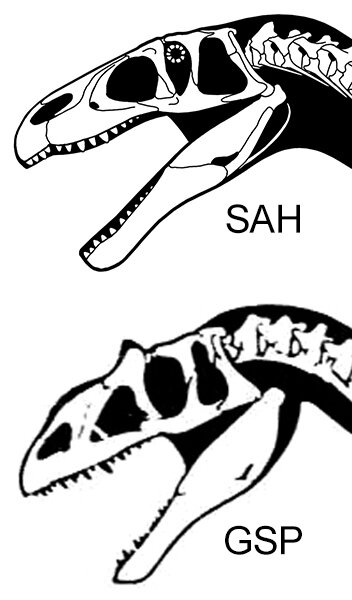This black-and-white illustration features two detailed profiles of dinosaur skulls labeled "S-A-H" and "G-S-P." Positioned one above the other, both skulls are depicted facing left, showing the nasal and eyeball cavities, jaws, teeth, and part of the spine. The top skull (S-A-H) is clearer and showcases larger, white-colored teeth, while the bottom skull (G-S-P) appears fuzzier, with smaller, black-colored teeth. Both dinosaurs have their mouths open, displaying variations such as a small circular detail on the top skull and a ridge near the eye on the bottom one. Despite these differences, the overall structures suggest a similarity, reminiscent of raptors, adding an element of predatory dinosaur-like Velociraptors from the Jurassic era.